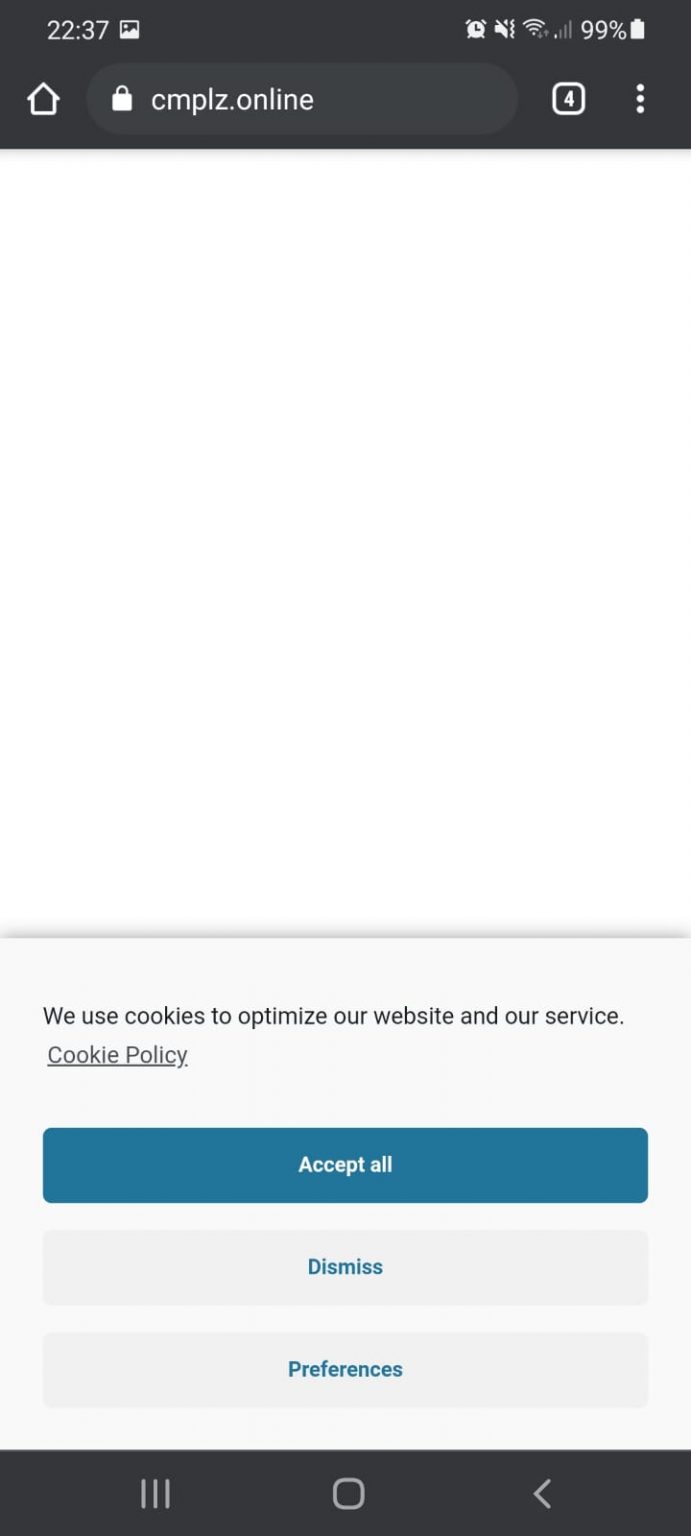**Descriptive Caption:**

The image appears to be a screenshot of a website taken on a mobile device. In the top right corner, there is a vertical white battery icon that is full, indicating a 99% battery level, which is displayed next to it. To the left, there's a phone signal strength icon at 1 bar, adjacent to a Wi-Fi signal strength icon at 4 bars. Further left, there's a muted sound icon with a slash through it and an alarm clock icon. On the top left, the time is displayed as "20:20," with a small photo icon to its right.

Directly below these icons, the URL bar shows "cmplz.online" in white text, with a white square containing the number 4 to its right. At the bottom of the image, there are three white horizontal lines on the left, a white square to their right, and an arrow pointing left even further right.

In the lower part of the image, a notification box is displayed, stating: "We use cookies to optimize our website and our service." Below this, the text "Cookie policy" is visible with an underscore line. Underneath, there are three buttons labeled "Accept All," "Dismiss," and "Preferences."